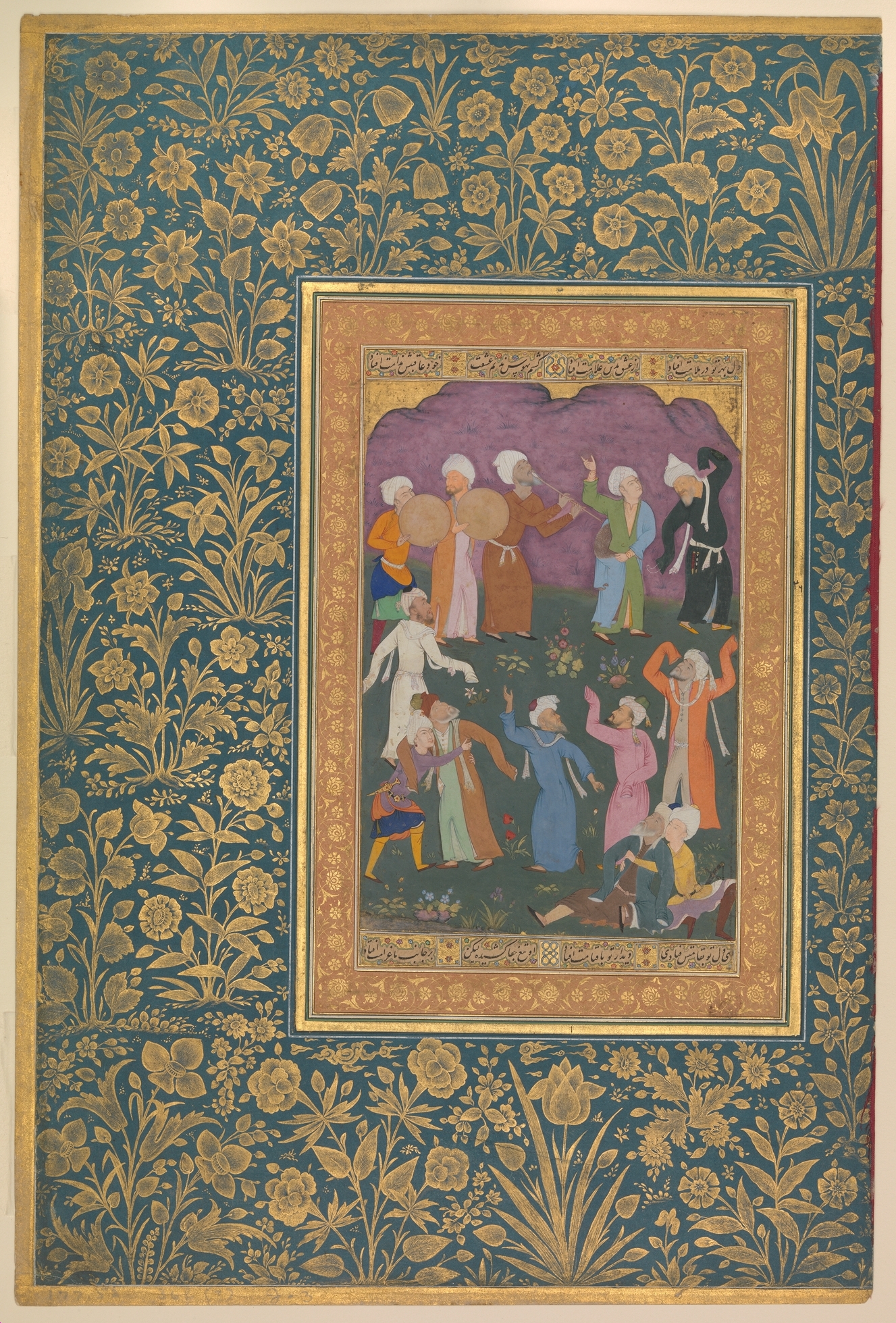The image is an intricate painting set against a background that resembles dark turquoise or bluish-gray wallpaper adorned with a gold floral pattern. The central painting, bordered by a yellowish-gold frame, depicts a lively celebration. Inside this ornate frame, smaller proportions mirror the same decorative themes, including a hint of the green background in its borders. The painting itself features numerous people dressed in traditional garb with vibrant colors including black, green, orange, brown, red, and blue. These individuals, portrayed in a cartoonish manner, seem to be joyous and animated, with many raising their hands in the air. Some participants are dancing and others are playing musical instruments like woodwinds and tambourines, while a few are sitting on the ground. The scene suggests a festive gathering, possibly with hints of grassy areas and a distant purple backdrop that could be interpreted as mountains. The characters, possibly including both men and women of varying ethnicities, are dressed in traditional long robes, enhancing the image's old-school charm and cultural richness.